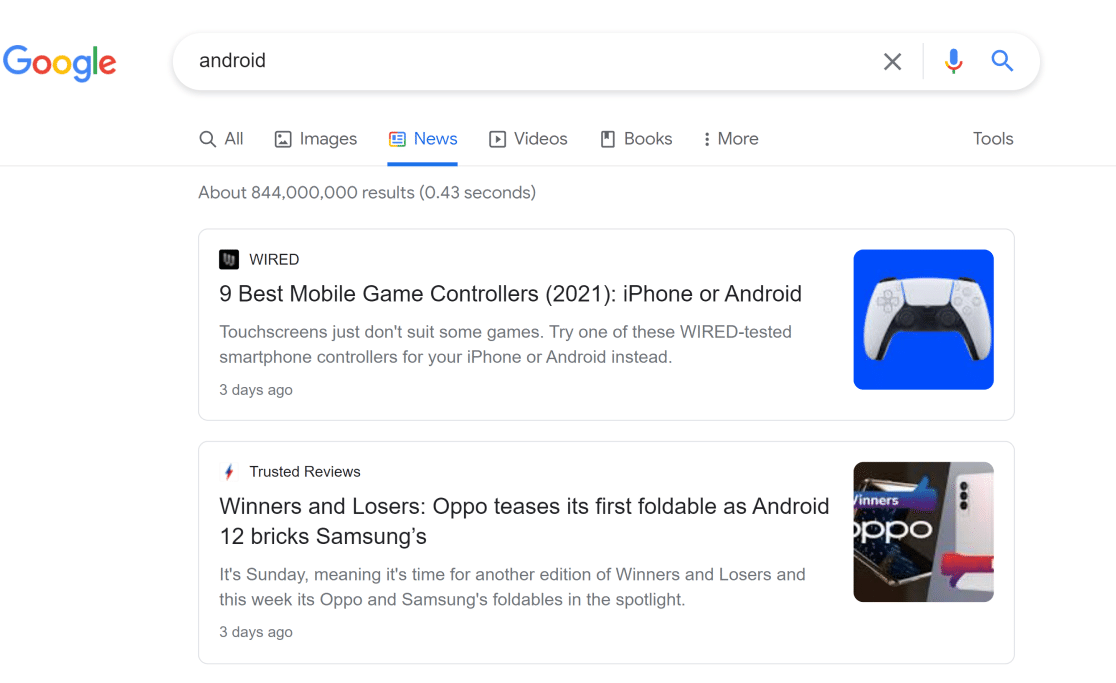A detailed screenshot of a Google search results page reveals the query "Android" has been entered into the search bar visible at the top. Dominating the top left corner, the recognizable Google logo signifies the platform. Positioned adjacently, the search query "Android" is clearly displayed, with the "News" tab highlighted in blue beneath it.

The search results boast about 844 million findings, achieved in a swift 0.43 seconds, as noted below the search query. The results feature two notable articles encased in distinct rectangular borders.

The primary result, sourced from Wired, spotlights their logo in the upper left corner of the box. The article headline, "9 Best Mobile Game Controllers 2021: iPhone or Android," is prominently displayed, accompanied by an image of a game controller on its right.

The secondary article, provided by Trusted Reviews, presents a headline titled "Winners and Losers: Oppo Teases its First Foldable as Android 12 Bricks Samsungs," along with their logo and a "Winners Oppo" logo. To the right, an image of a smartphone subtly augments the article’s appeal.

This screenshot encapsulates a comprehensive view of Google's efficient and expansive search results for the term "Android," highlighting pertinent tech news from reputable sources.